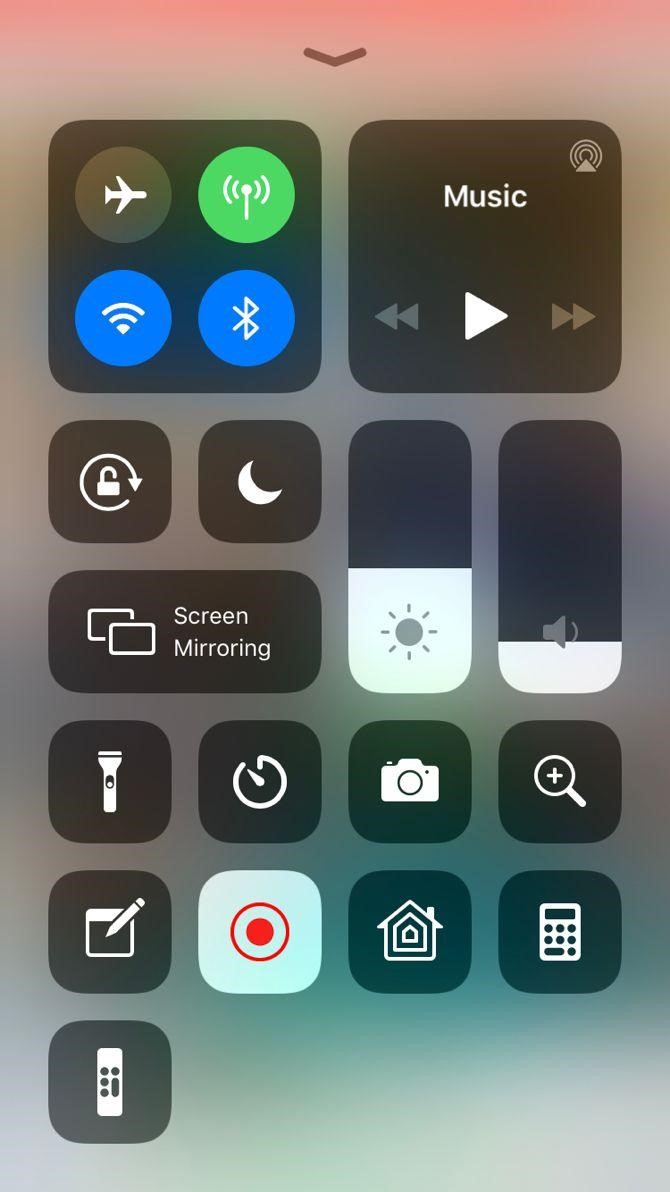In this image, we are looking at a screenshot of a cell phone's control center interface. The background features a very muted and abstract color gradient. At the top, it transitions from a pinkish tone mixed with ivory down to grays and taupe, ending in pale ivory green towards the bottom of the screen.

At the top section of the screen, there are several black circular icons. Starting from the left, we see icons for Airplane Mode, Cellular Data, Wi-Fi, and Bluetooth. To the right of these icons, there is a box designated for music controls, featuring 'Music' in white text alongside a play button that is highlighted.

Below this row, there is a black button featuring the 'Do Not Disturb' Moon icon. Directly beneath that, there is a rectangular button labeled 'Screen Mirroring'. Continuing downwards, on the bottom-right corner, there is a button for the calculator, while on the bottom-left corner, there is a house icon representing the Home button.